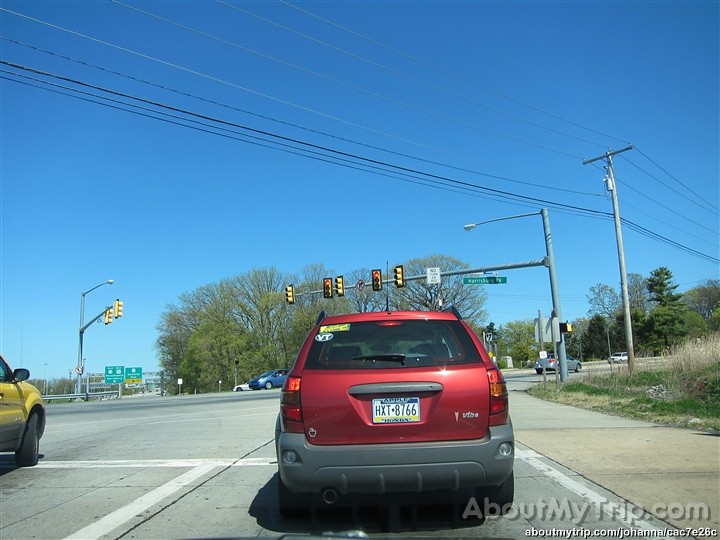This vibrant color photograph captures an outdoor scene viewed from inside a car through the windshield. The composition includes a red SUV prominently positioned at the center bottom, parked at a traffic light intersection. The asphalt, illuminated by the bright sunlight, appears light gray. On the left side, a road or highway adorned with green directional signs arcs gracefully into the background. The surrounding landscape is rich with greenery, featuring lush trees and scattered vehicles, adding life to the scene. Enhancing the image is a translucent logo in the bottom right corner that reads "aboutmytrip.com," with the website address in smaller text below. The scene radiates the warmth and clarity of a bright, sunny day, suggesting an inviting and picturesque journey.